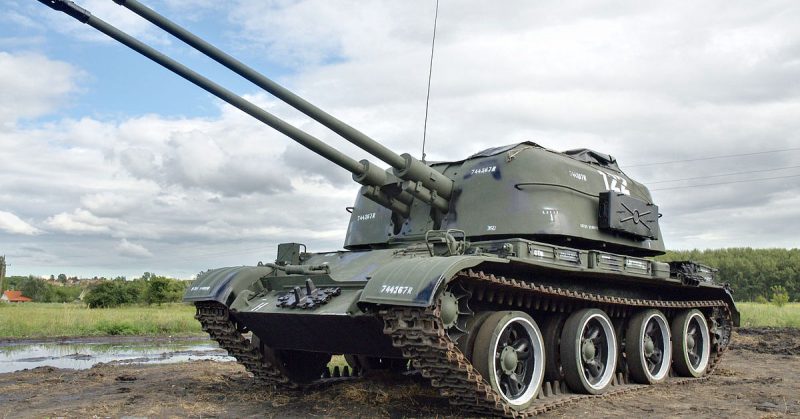The image depicts a large, dark green military tank with distinctive features. It is situated in a muddy field, with puddles indicating recent rainfall. The tank has four wheels visible on the side, encased in tank treads. This serves as part of its robust mobile artillery system. Notably, the tank is equipped with two side-by-side cannons protruding from the front, an unusual feature for typical tanks that often have a single cannon. Numbered markings are visible in various places on its surface, including the number "122" in white lettering prominently displayed on the side, and possibly "7442672" on other parts of the tank. An antenna extends from the top, which appears capable of rotating, though it is currently oriented forward. The scene is set during an overcast day, with a mostly cloudy sky accented by patches of blue. In the background, beyond the muddy area, there is a field of tall grass leading to a distant tree line, and a house with a red roof is faintly visible to the left.